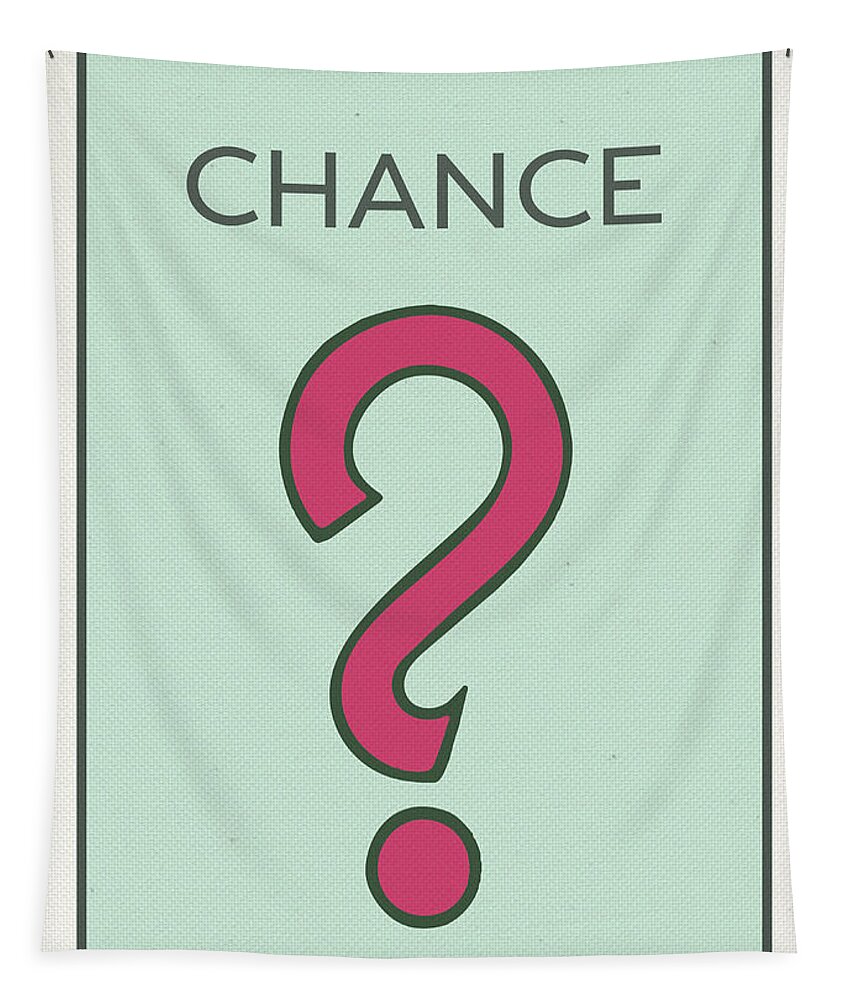This is a detailed description of a banner from the game Monopoly, featuring a design reminiscent of canvas fabric with a light spring green background. The banner is bordered by two black vertical lines on the left and right edges, with the top and bottom edges cut off, possibly suggesting it's part of a larger image or box. At the top, there are bold black letters forming a word or phrase, although the exact text is not specified. Dominating the center of the banner is a large red question mark, intricately designed with a curly tail and outlined in black. The question mark extends from the top center down to the bottom, ending with a prominent dot. The banner appears to be draped in a slight U-shape, suggesting it is loosely hung, possibly by nails that are just out of view at the top left and right corners. The material, likely canvas or fabric, adds to the textured, vintage aesthetic of the piece.